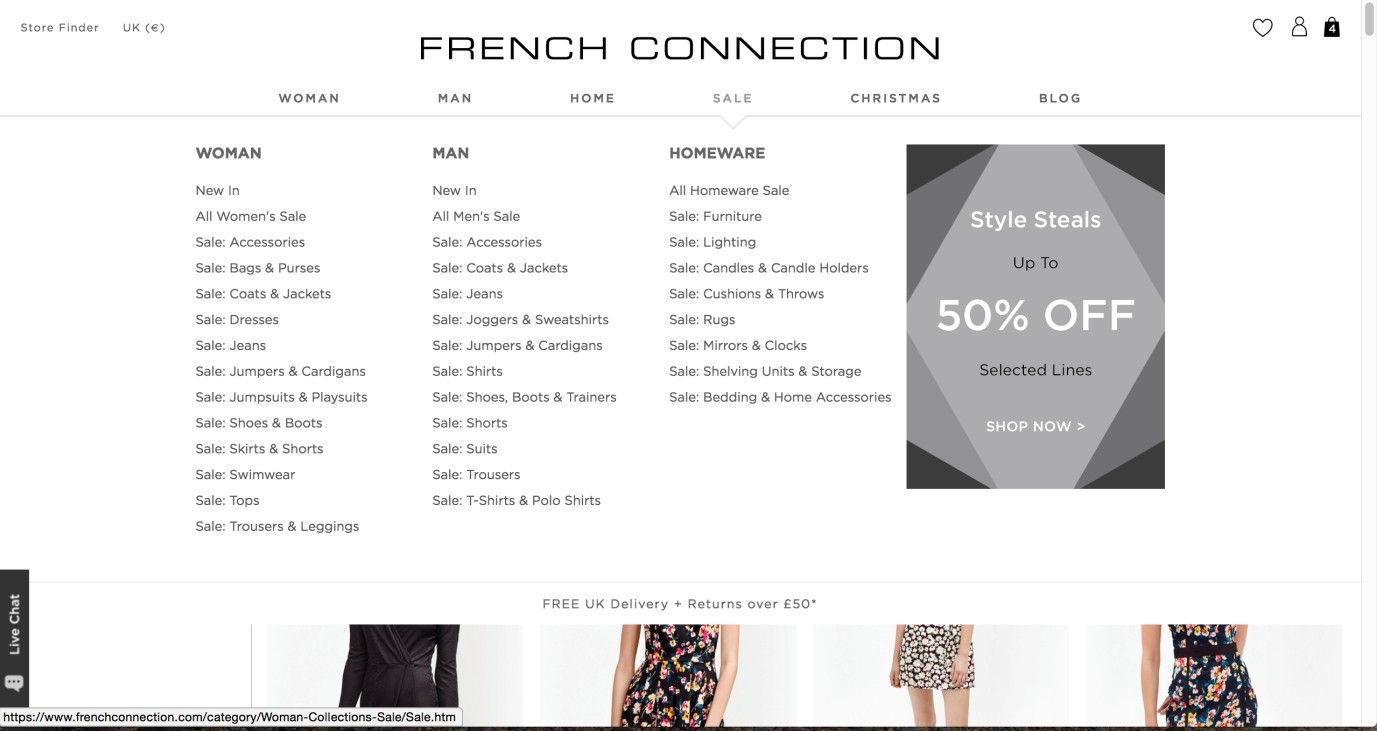The image depicts a sleek, predominantly white webpage for the French Connection retail brand. At the center, the brand name "French Connection" is prominently displayed in elegant black text. The webpage features an intuitive navigation bar with multiple options, including "Store Finder" and regional selection options such as "UK." 

Various functional icons are lined up at the top right corner, including a heart symbol for favorites, a person symbol for user account access, and a shopping bag icon displaying the number '4,' indicating four items presently in the shopping cart.

The navigation menu is structured to include categories such as "Women," "Men," "Homepage," "Sale," "Christmas," and "Blog." A highlighted banner announces an enticing offer: "Style Steals Up to 50% Off Selected Lines. Shop Now." 

Under the "Sale" tab, sub-sections include "New In," "All Women's Sales," and other assorted categories detailing the items available at discounted prices. Further down the page, images showcase select women's clothing items, including elegant black floral dresses and professional suits, emphasizing their inclusion in the sales collection.

Additionally, a live chat button in black is available for immediate assistance. The URL of the website is visible at the bottom, confirming it as a shopping site. This well-organized webpage is designed to facilitate a seamless online shopping experience with a clear, detailed layout.